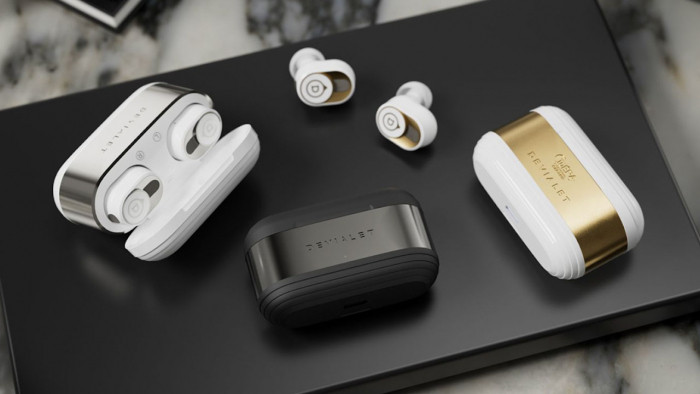The indoor scene features a white marble countertop with gray veining in the background, atop which rests a slim, matte black rectangular object, possibly a laptop or pad. Centered on the black surface are three sleek, oval-shaped wireless earbud cases. The case on the lower right is white with a gold trim, its lid open to reveal the bulky, gold-trim-wired earphones nestled inside. To the left, a black matte case with a black band lies closed, while in the upper left corner, a white case with a silver trim holds its contents securely shut. Above the black surface, two white earphones with gold interiors rest loose, showcasing their elegant design. The image emphasizes a luxurious and high-end aesthetic for these cutting-edge technology instruments.